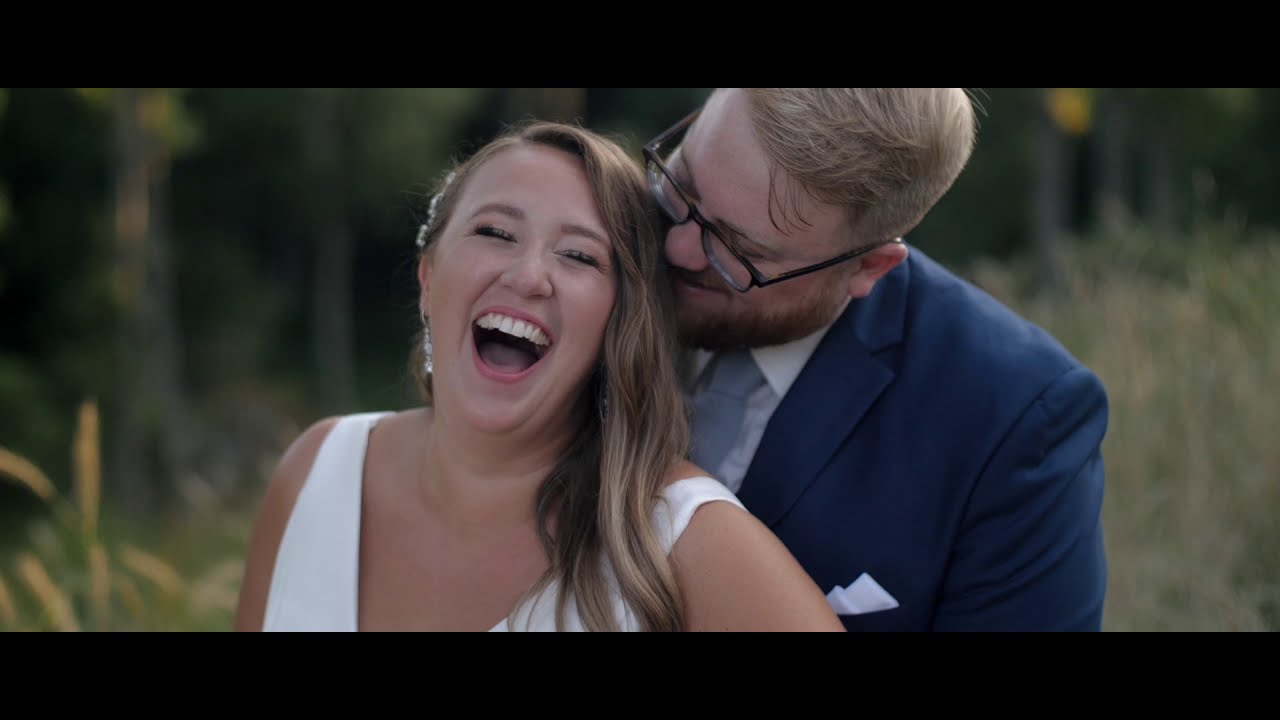In this professional outdoor wedding photograph, a newlywed couple is captured in a tender moment. The man, with his blonde hair and orange beard, is wearing a blue suit, white shirt, blue tie, and sports a pair of glasses. He stands behind his bride, leaning over to kiss her on the head. His suit is complemented by a white pocket square. The bride, donning a white wedding gown with short sleeves, has her long, half-blonde, half-brown hair elegantly styled to one side and adorned with white beads and flowers. She is smiling widely, her eyes closed in joy, showcasing her lipstick and diamond earrings. The couple is surrounded by a picturesque outdoor setting with lush green grass, trees with full foliage, and marsh plants, all slightly blurred to emphasize the pair’s joyous expressions. The image itself is bordered by black rectangular bars on the top and bottom, adding a cinematic touch to their beautiful moment.